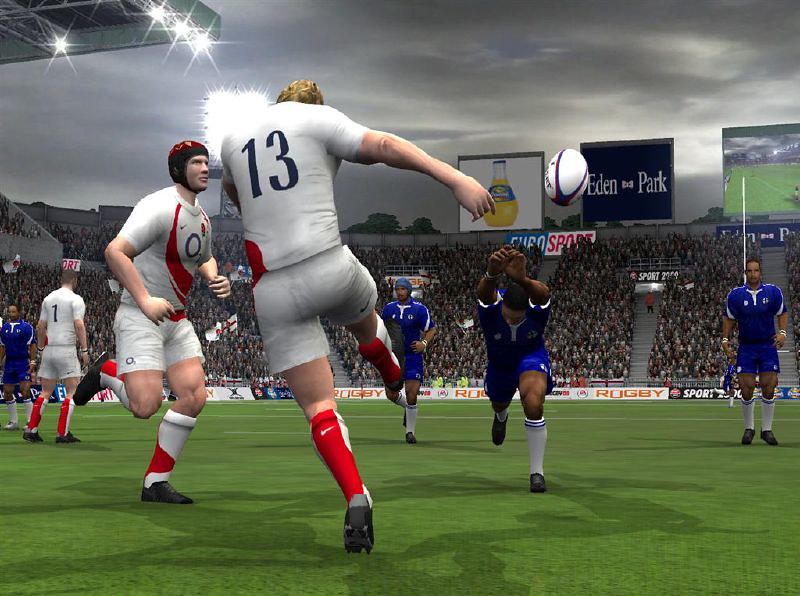The image is a highly realistic rendering resembling a video game scene. It depicts a dynamic moment in a rugby match, set in an open-air stadium with a crowd of spectators. The field is a vibrant green, surrounded by stands filled with fans. Various players are captured mid-action, their attire distinct: some wear blue jerseys with white trim, blue shorts featuring a similar white trim, and white socks with blue stripes, while others are clad in white jerseys, white shorts, and red-and-white socks. All the players sport dark-colored low-top shoes. In the air, a rugby ball, predominantly white with blue lines and some red detailing, is suspended between the vying players. The stadium’s promotional signage reads "Eden Park," indicating the venue, while another sign mentions "sport" in white letters on a black background. The sky above the stadium exhibits a twilight blue hue with some cloud cover, suggesting an evening setting.